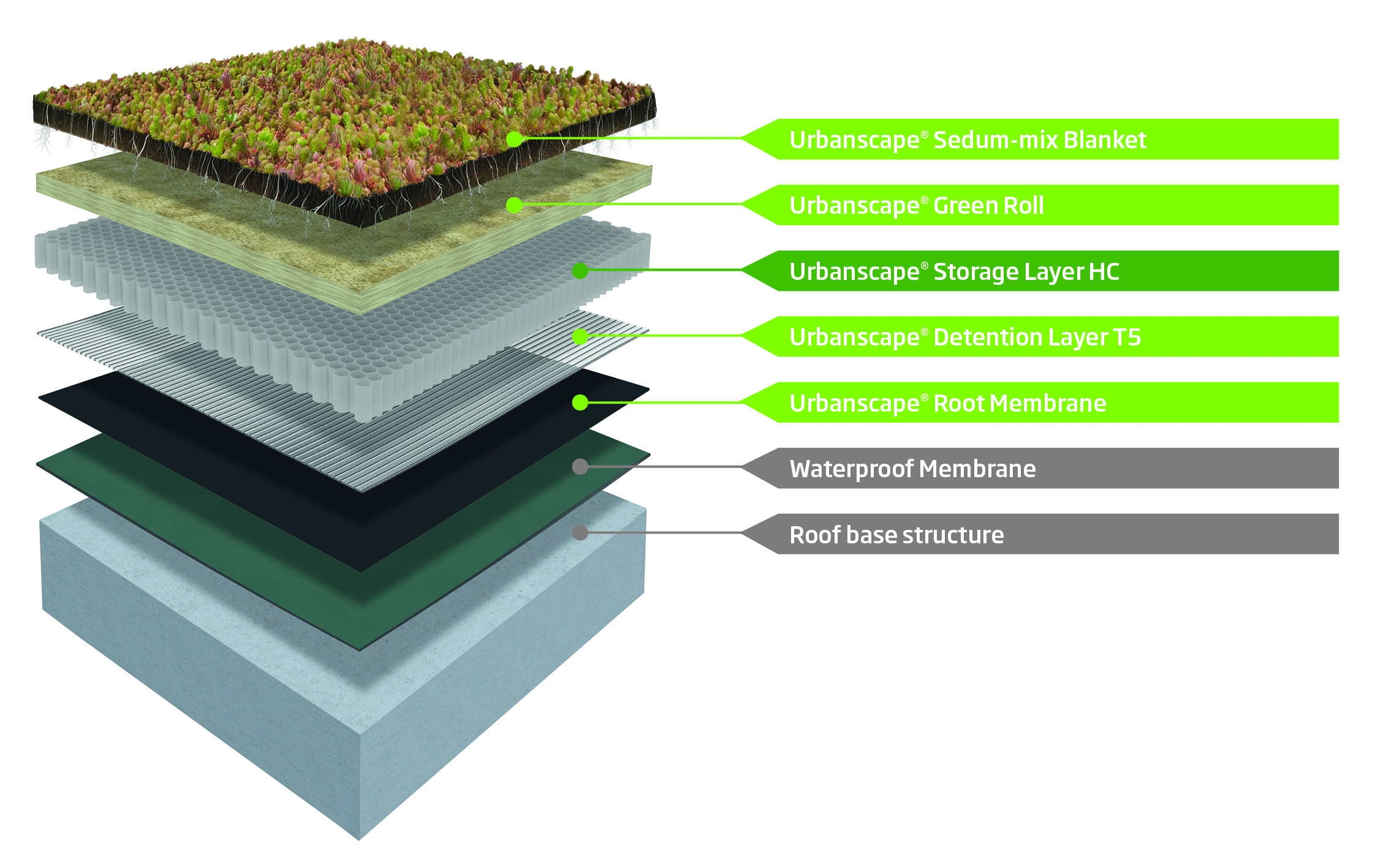The image is a detailed diagram illustrating the cross-section layers of an outdoor roofing system. Positioned at an angle, the layers resemble overlapping squares. Each layer is labeled with descriptive text to the right of the diagram. At the topmost layer, some small green plants and a reddish plant are visible, cultivated on a black tray labeled "Urbanscape Sedum Mix Blanket." Below this, a green arrow points to the "Urbanscape Green Roll." Continuing downward, a dark green arrow indicates the "Urbanscape Storage Layer HC," followed by another light green layer labeled "Urbanscape Detention Layer T5." Further down, there is another light green layer marked as "Urbanscape Root Membrane." The subsequent gray layer is identified as the "Waterproof Membrane." Finally, the bottom layer, depicted in a light blue or cement grey color, is labeled "Roof Base Structure." Each label is written in white text on either green or gray arrows.